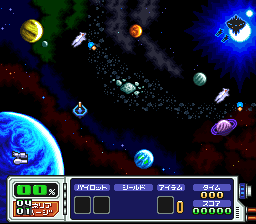A detailed screen capture of a mobile outer space video game, showcasing a vibrant and dynamic cosmic scene. In the background, a dark expanse of space with layered colors of black, blue, red, and green is dotted with twinkling stars in blue and orange. There is a bright white star glowing blue in the distance. Off to the side, a yellow and black planet can be seen, along with a blue Earth-like planet with white swirls of clouds.

In the upper right corner, a large spaceship is visible, appearing to launch two smaller spaceships that are heading towards the Earth-like planet. These spaceships seem to be part of a shooting sequence in the game. Scattered throughout the scene is an asteroid belt composed of numerous rocks, adding to the space ambiance. A small spaceman is also flying in the vicinity, contributing to the action-packed environment of the game.

At the bottom of the image, there is a box displaying text and numbers that appear to be in Japanese, most likely indicating the player's score and health. The indicators and score lines are in a variety of colors, including orange, white, purple, yellow, and green, accentuating the intricate interface of the game. The numeric displays include sections showing "zero percent health" and a score count, emphasizing the game's competitive elements.